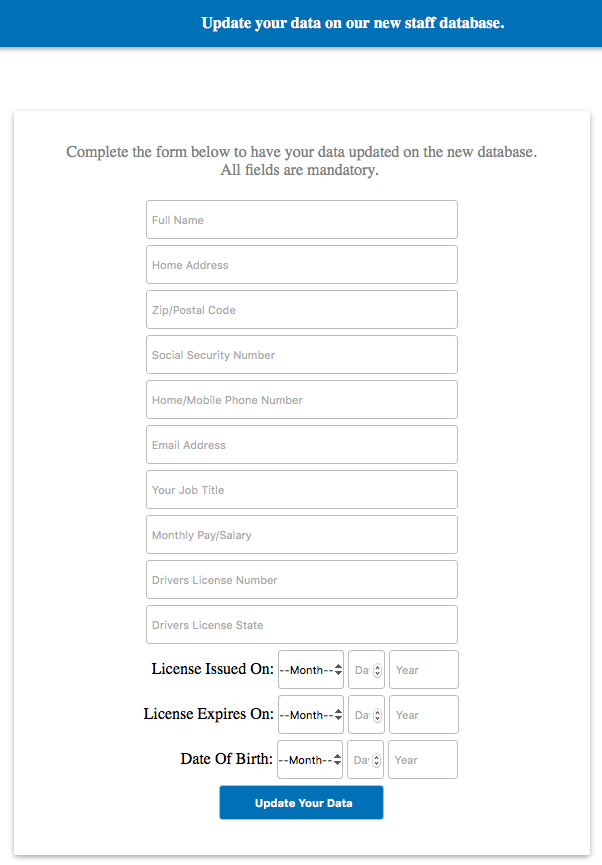In the image, there is a predominantly white page featuring numerous input fields designed for updating data. The text is mostly black, with some elements in gray, enhancing readability. At the top of the page, a blue bar prominently displays the message: "Update your data on our new staff database."

Directly below the bar, a concise instruction reads: "Complete the form below to have your data updated on the new database. All fields are mandatory."

The form includes the following sections for user input:
- Full Name
- Home Address
- Zip/Postal Code
- Social Security Number
- Home/Mobile Phone Number
- Email Address
- Job Title
- Monthly Pay/Salary
- Driver's License Number
- Driver's License State

Further down, the form has additional boxes for filling in specifics about the driver's license:
- License Issued On (with separate boxes for Month, Day, and Year)
- License Expires On (also with separate boxes for Month, Day, and Year)
- Date of Birth (with separate boxes for Month, Day, and Year)

At the bottom of the form, a blue button labeled "Update Your Data" is visible, which users are presumably required to click to submit their filled-in information for processing and confirmation.